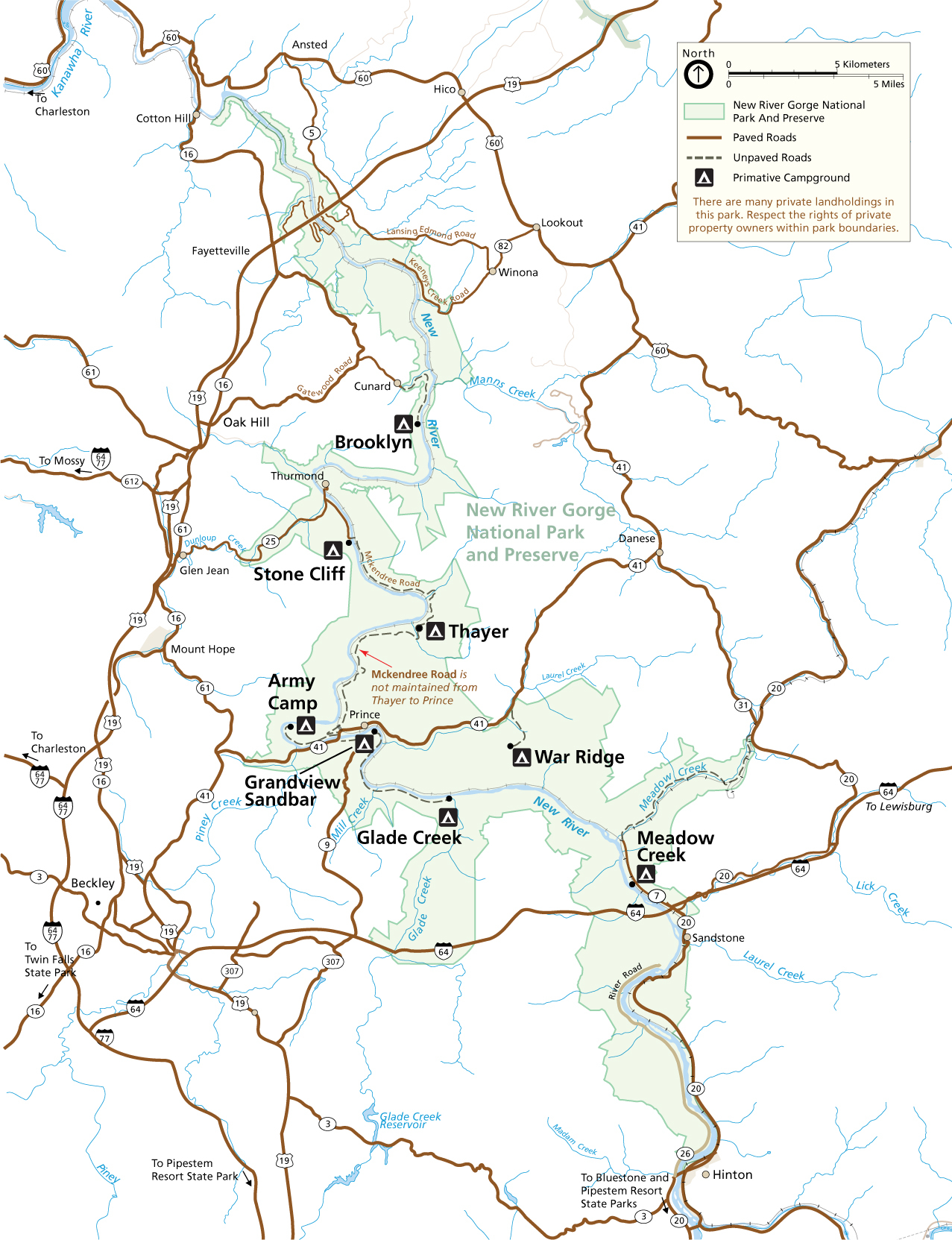This detailed map features a diagram in the top right corner showing a scale in kilometers and miles, accompanied by a north arrow within a black circle. A legend in this key explains various symbols and lines: a black line for distance, a light blue rectangle indicating "New River Gorge National Park and Preserve," a solid line for paved roads, a dotted line for unpaved roads, and a black box with a white triangle representing primitive campgrounds. It notes the presence of private landholdings within the park. The map has a white background with roads in brown, blue areas depicting bodies of water like creeks and rivers, and green areas for natural features. Various locations such as Brooklyn, Stonecliff, Thayer, Army Camp, Grandview Sandbar, Great Glade Creek, Warridge, Meadow Creek, and Beckley are marked. The map includes numbered highways and has detailed labels for waterways and campsites, emphasizing the extensive network of roads and pathways throughout the park.